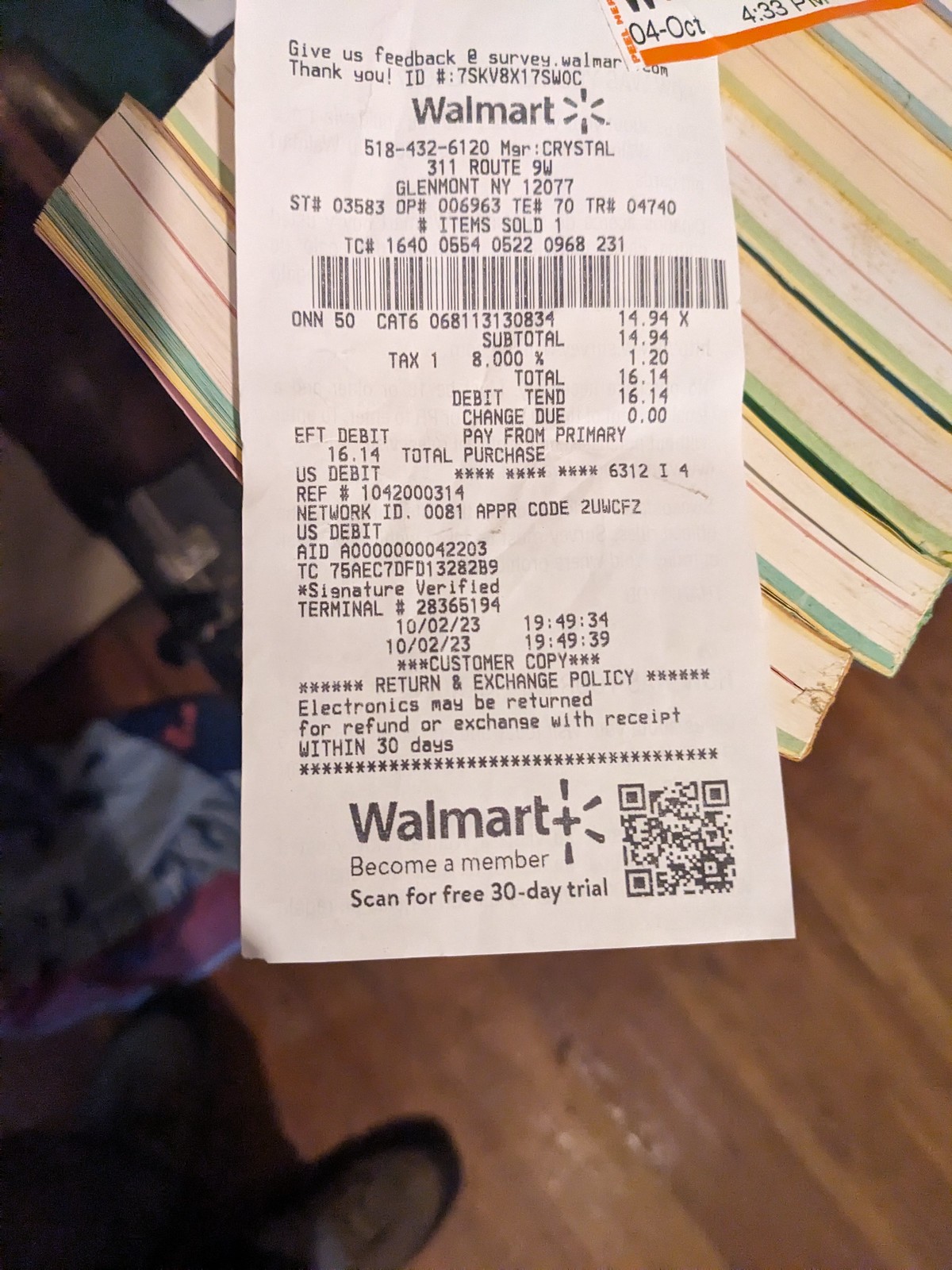This detailed photograph captures a Walmart receipt from the Glenmont, New York location, set against the backdrop of a person's foot visible in the background. The receipt is either being held by the individual or placed atop a stack of books that rest on a desk or table. The purchased item is not entirely clear but includes a description "O-N-N 50 cat" priced at $14.94, which totals to $16.14 after tax. Payment was made via debit card, and the receipt includes extensive store identification details along with a "Signature Verified" terminal number. The transaction date is October 2nd, 2023, specifically at 19:49 (7:49 PM). At the bottom of the receipt, there is a promotional message encouraging new membership with a 30-day free trial, accompanied by a QR code for easy access.